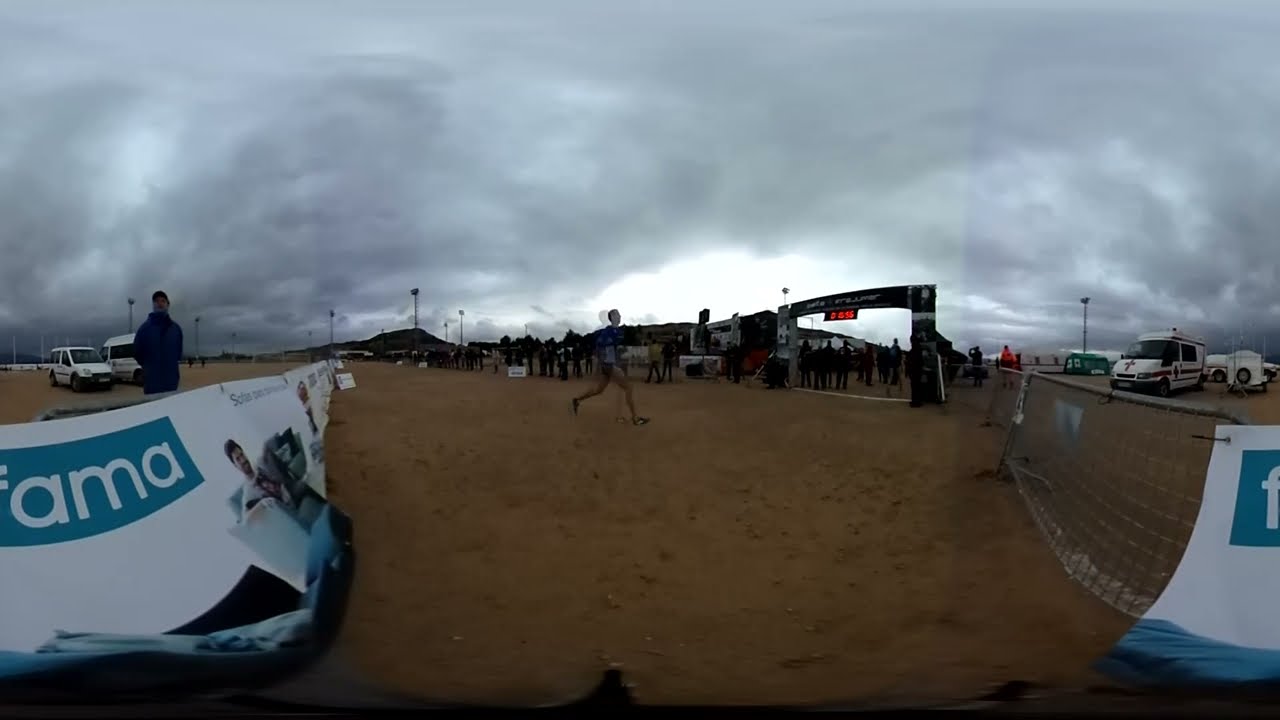This image captures the entrance to an event under a somber, overcast sky filled with gray and black clouds. In the foreground, a sandy, dirt area leads to a series of netting fences that direct cars towards a domed, possibly temporary, graphite-constructed entrance crowned by a digital sign. European-style vehicles populate the scene, including two white vans parked on the left and an ambulance with a red cross on the hood stationed in the center-right. Groups of people congregate and line up in front of the camera, adding to the bustling atmosphere. A metal fence to the right and an advertising billboard railing to the left further frame the scene. The right side background features a lineup of mostly white cars, reinforcing the European setting. Lights, though present, are not illuminated, leaving the area under the muted natural light from the cloud-covered sky.